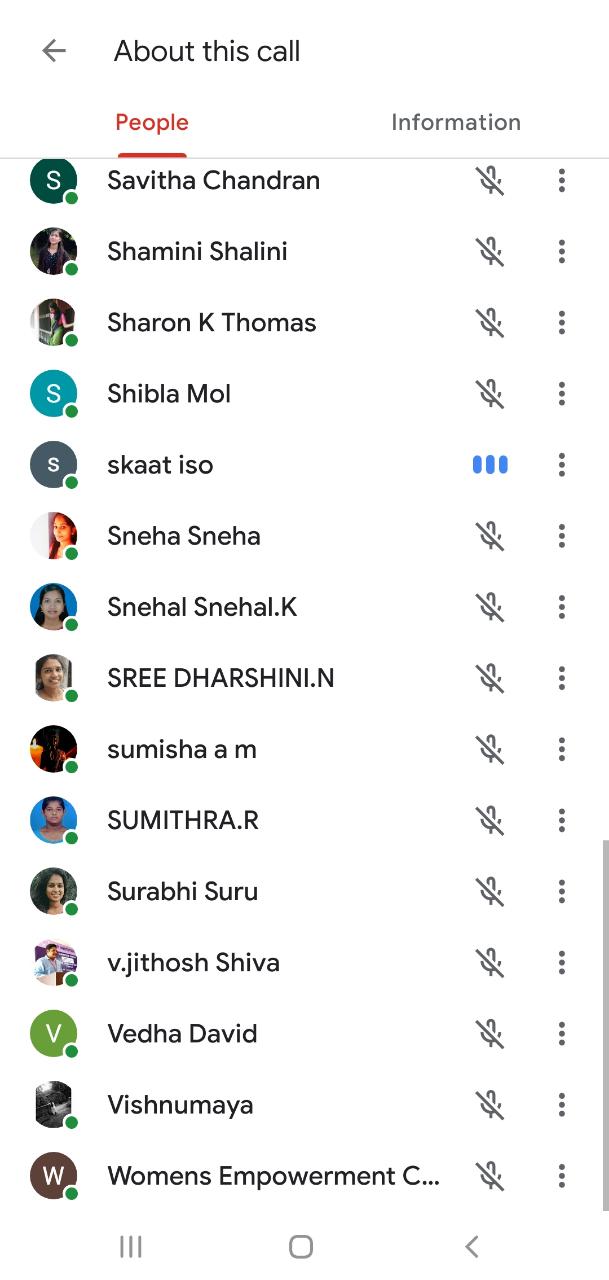This image is a detailed screenshot of a user's phone displaying their contact list, labeled "About This Call" at the top. Just below this title, there are two tabs: the "People" tab, which is highlighted in red, and the "Information" tab, which appears in grey. The main list beneath these tabs features several contacts. On the left side, each contact is accompanied by an avatar—mostly photographs of people's faces—with a small green dot on each, indicating that they are currently online. On the right side, each contact has a microphone icon next to their name, except for "Skart Eso," which is distinguished by three blue dots instead of the microphone emblem. This intricate setup offers a clear and structured overview of the user's contacts and their online status in the context of an ongoing call.